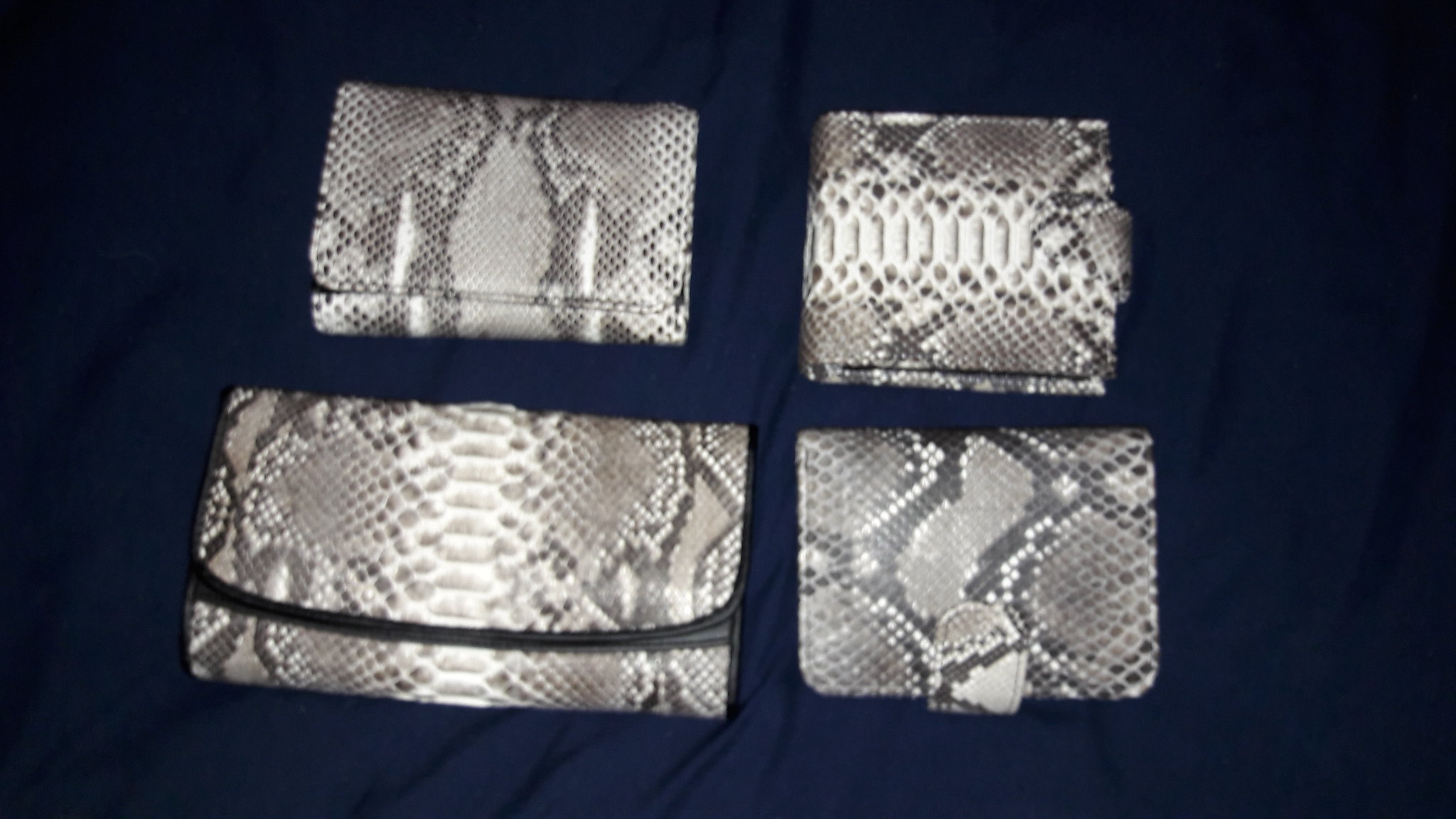Displayed against a blue material backdrop, the photograph captures a top view of four distinct clutches and wallets arranged in a square. Each item features a textured, snakeskin pattern in varying shades of grey, black, and white. The top left item is a sophisticated clutch with a fold-over design, embodying a sleek appearance. To its right, there is a compact bifold wallet with a visible clasp on its right side. The bottom left showcases the largest piece, a spacious clutch that folds down from the top, reinforced with black leather rims for a striking contrast. Finally, the bottom right item is another clutch, bearing similarities to the bifold wallet with a clasp at its bottom. Each piece shares a common snakeskin design, yet they differ in shape and closure style, providing a unique but cohesive collection.